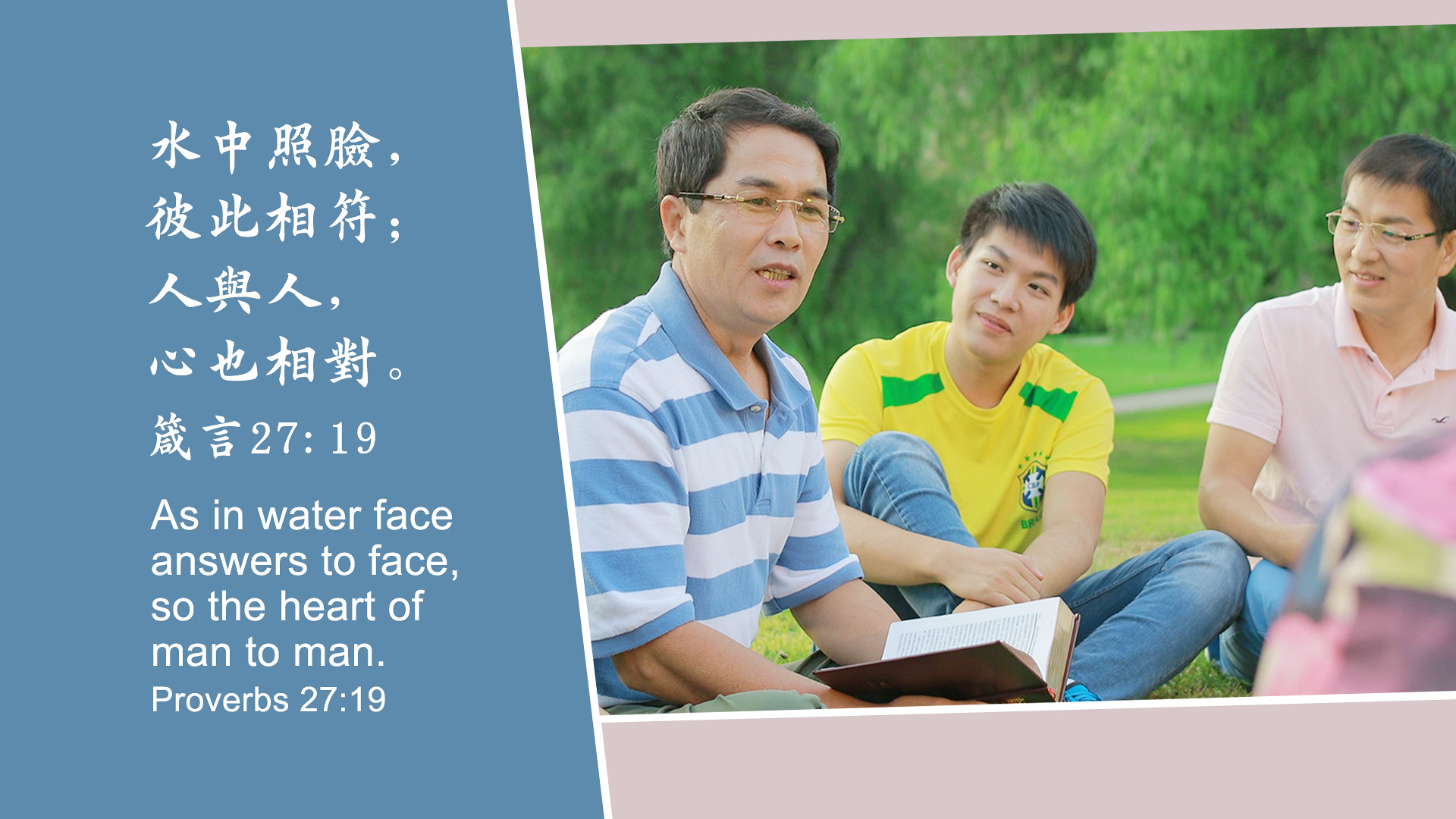This landscape-oriented image depicts a scene likely related to a Bible study. The photo is set against a blue background on the left third, which features both Chinese (or Japanese) text and an English translation of Proverbs 27:19: "As in water face reflects face, so the heart of man to man." A thin white pinstripe separates this section from a photograph taking up the right two-thirds of the image.

In the photo, three Asian men are seated on grass, framed by the lush green of surrounding trees. On the far left, an older man with glasses and hints of gray in his black hair is focused on an open book in his lap, probably a Bible. He is dressed in a blue and white striped polo shirt. Next to him, a younger man in a yellow short-sleeved t-shirt with green stripes on the shoulders and blue jeans gazes intently at him. The third man, positioned on the right, wears a pink polo shirt and glasses, his attention also directed towards the central figure. The image is bordered by light pink headers and footers, adding a soft contrast to the overarching theme of reflection and study.